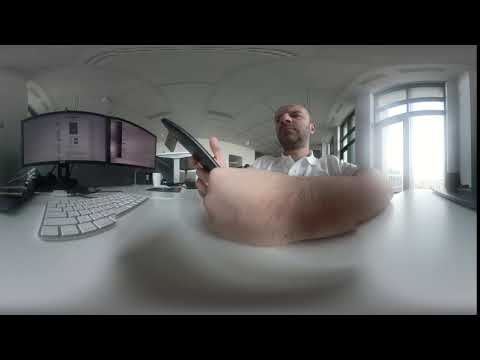In this photograph, a balding white man with pale skin and a beard is seated in a modern office setting. He is wearing a white polo shirt and appears to be interacting with a black smartphone. His posture is casual, with one arm resting on a white desk, resembling a distorted foot due to the wide-angle lens used in the image. The desk holds a white and gray computer keyboard and two black monitors, currently displaying white web pages.

The office has a white ceiling and multiple rooms visible through doorways or windows behind him. These large windows, with dark gray frames, stretch from floor to ceiling, allowing bright light to flood the space. To the left side of the room, there is a gray mezzanine or balcony-like structure. The overall image has a fisheye effect, adding to the sense of distortion. The photograph captures a blend of natural and artificial light, contributing to the airy and spacious feel of the office.